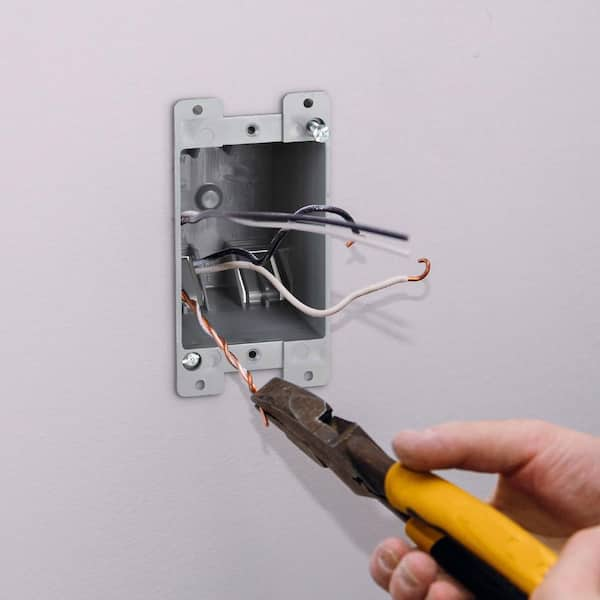The photo is a close-up color image of an electrician performing electrical work on a wall-mounted electrical workbox. The workbox, which is square and secured with screws, is embedded in a light gray wall. The electrician's right hand is visible, grasping a pair of somewhat aged, yellow and black insulated pliers with a square tip and built-in cutters. The electrician is twisting a pigtail connection—a method to join multiple wires in the workbox. The wires are clearly visible: white for the common, black for the hot, and a copper ground wire. The pigtail connection is being made with the copper ground wire, held firmly by the pliers. Additionally, screws are protruding from the top right-hand corner of the box, indicating preparation for installing either an outlet or a light switch.